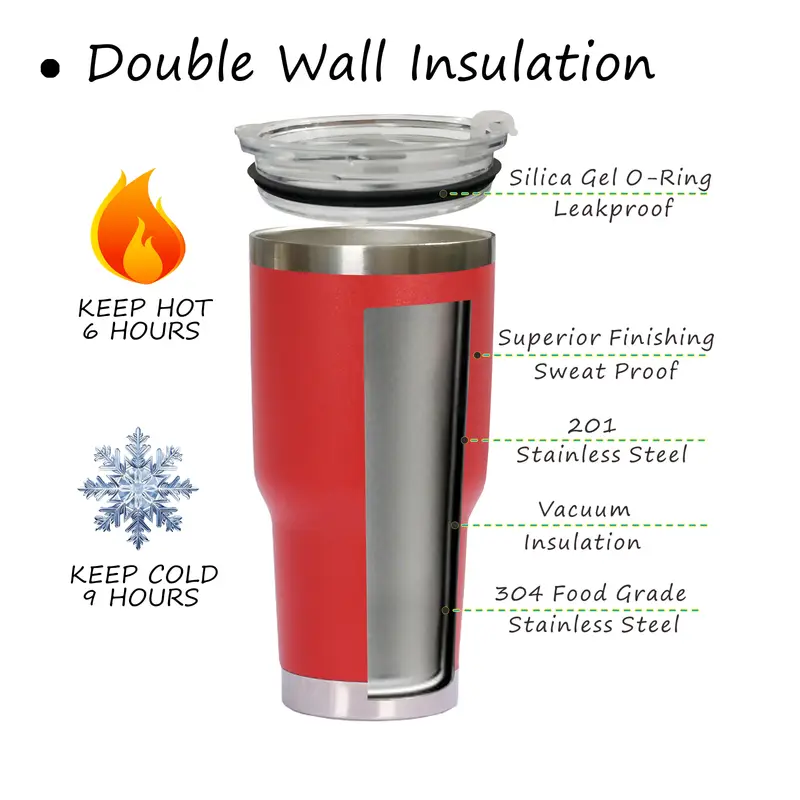The image is a detailed diagram of a red insulated tumbler against a white background. The tumbler features labels and illustrations highlighting its various qualities. At the top, in black text, it reads "Double Wall Insulation," with a bullet point featuring a black dot to its left. To the right, an illustration of flames in gradient colors—gold, orange, and yellow—indicates that the tumbler can "Keep hot for 6 hours." Below this, a blue and white snowflake signifies that it can "Keep cold for 9 hours."

On the right side, the diagram extensively labels the tumblers components and features. The top section depicts a transparent plastic lid with a black rubber band, labeled as "Silica Gel O-ring, Leak Proof." Further detailing the outer structure, labels point out "Superior Finishing, Sweat Proof" and "201 Stainless Steel." Inside, it showcases "Vacuum Insulation" and the innermost layer, "304 Food Grade Stainless Steel." The detailed depiction of the mug’s cross-section, including a gray interior and a silver bottom and rim, highlights its superior build quality and functionality.